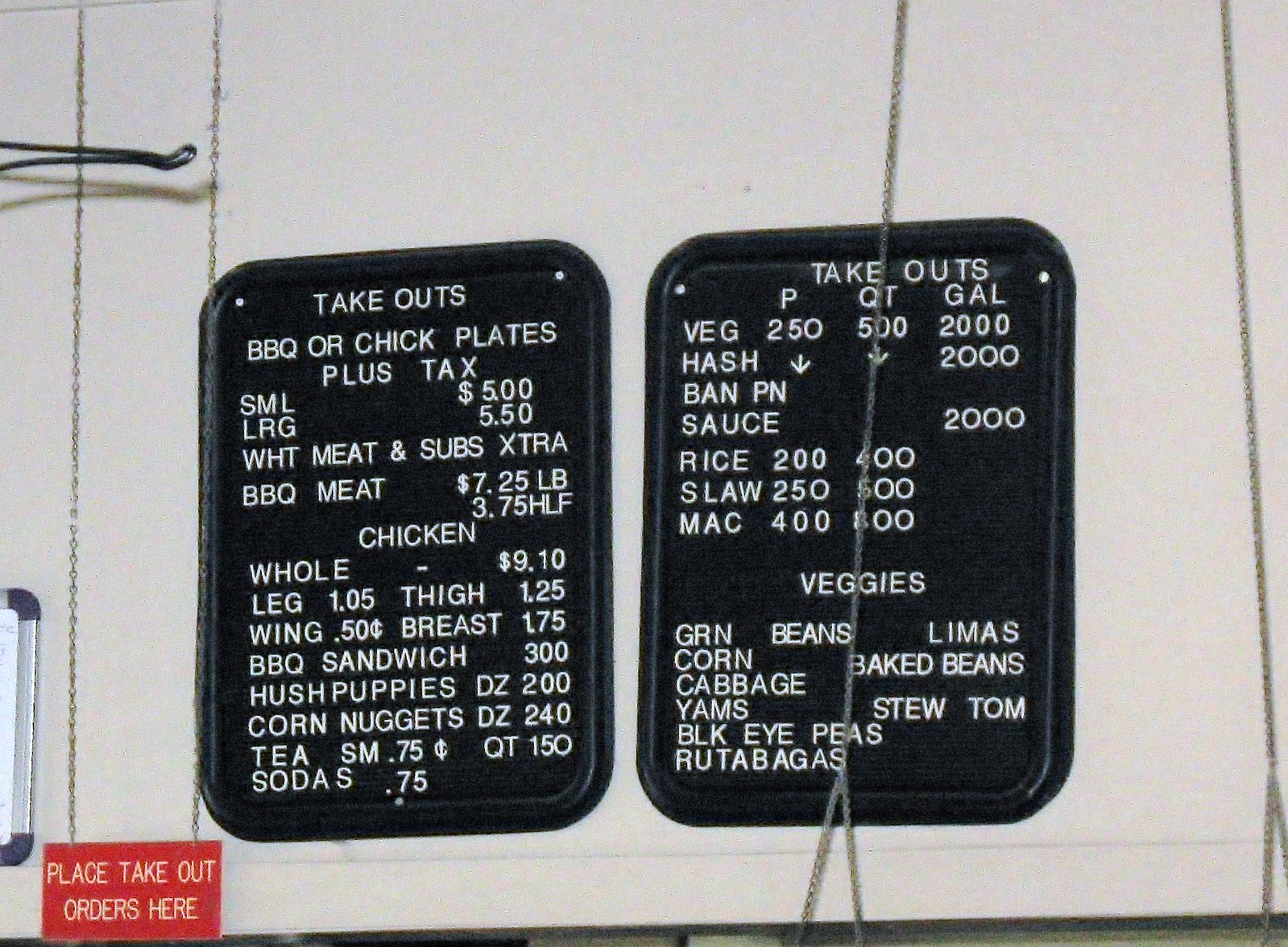The image features a detailed scene of a barbecue snack bar menu displayed on blackboards with white movable letters. The menu boards are suspended by chains on the left side, which also secure a sign indicating "Take Out Orders Here". A square whiteboard is prominently fixed on the wall, which is stark white and serves as a clean backdrop.

At the top of the wall, there's a small, curved metal structure hanging down, adding a rustic charm to the setting. The left blackboard lists a variety of barbecue items:

- **Take Out BBQ or Chicken Plates** (plus tax): Small $5, Large $5.50
- **White Meat Substitutes**: Extra BBQ Meat, $3.75 per half pound
- **Chicken**: Whole $9.10, Leg $1.05, Thigh $1.25, Wing $0.50, Breast $1.75
- **Barbecue Sandwich**: $3
- **Sides**: Hushpuppies (dozen) $2, Corn Nuggets (dozen) $2.40
- **Drinks**: Tea (small) $0.75, Quart $1.50, Soda $0.75

On the right blackboard, a variety of additional items are listed:
- **Vegetarian Options and Sides**: 
   - Hash
   - Banana Pudding
   - Sauce
   - Rice
   - Coleslaw
   - Mac and Cheese
   - Green Beans
   - Lima Beans
   - Corn
   - Baked Beans
   - Cabbage
   - Yams
   - Stewed Tomatoes
   - Black Eyed Peas
- **Ruler Vegas*** is noted at the bottom, although its meaning is unclear.

Below the menus, the opening for the takeout window is visible, where orders are likely placed and picked up. The setup exudes a classic, homely barbecue joint atmosphere.